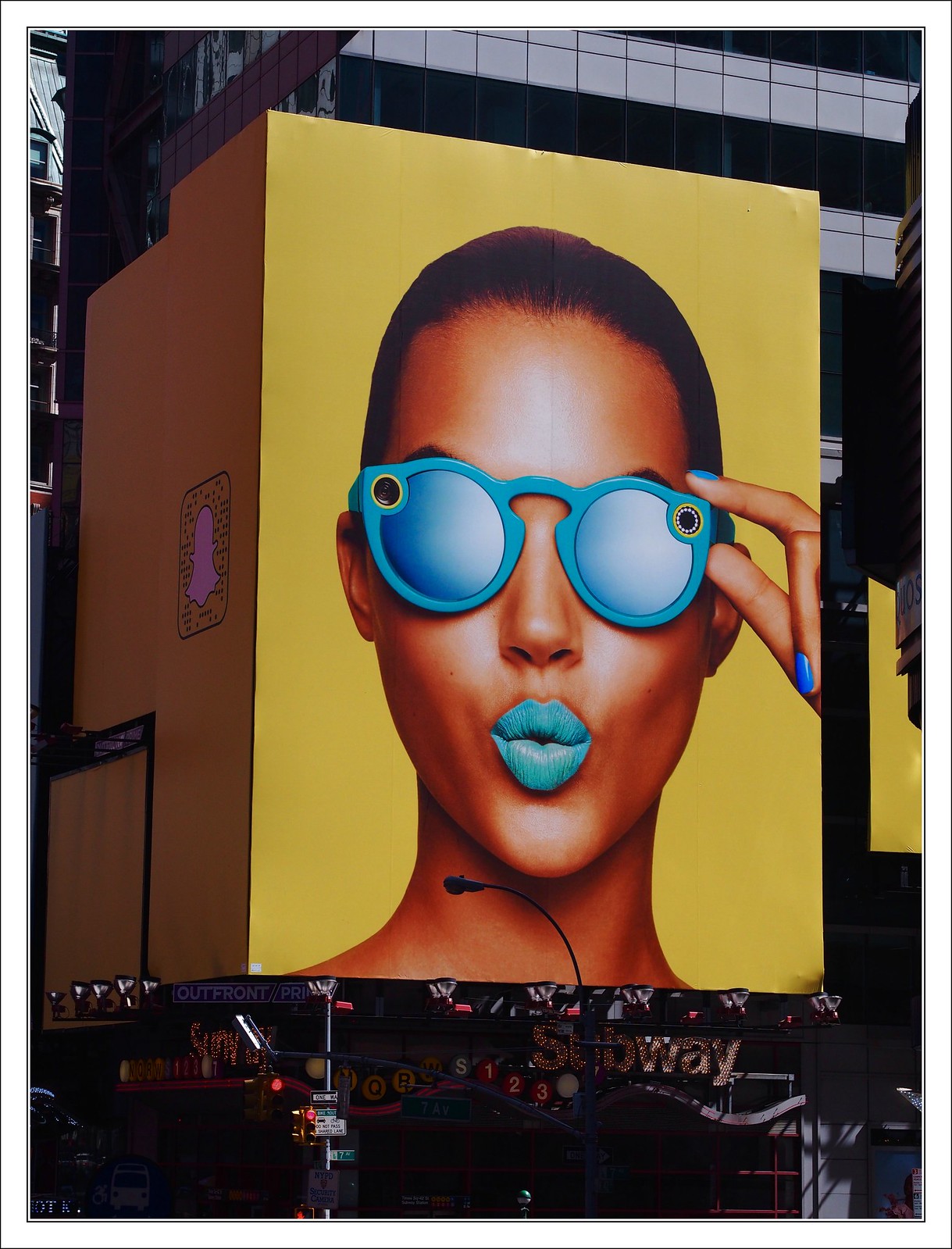The image depicts a large, vibrant billboard located in Times Square, promoting what appears to be a Snapchat filter. The principal focus of the advertisement is a close-up of a dark-skinned woman with her hair slicked back, possibly into a ponytail or bun. She sports striking blue cat-eye sunglasses that feature distinctive yellow circles with black centers on the corners of the frames, and her blue lips are pursed in a "kissing" expression. Adding to the monochromatic theme, she has matching blue fingernails and is seen holding the edge of her sunglasses with her right hand. The billboard's background is a bold yellow, enhancing the image's vivid look. Below this eye-catching advertisement, there is a black storefront that reads "subway," as well as various street signs, indicating the bustling cityscape setting of Times Square.